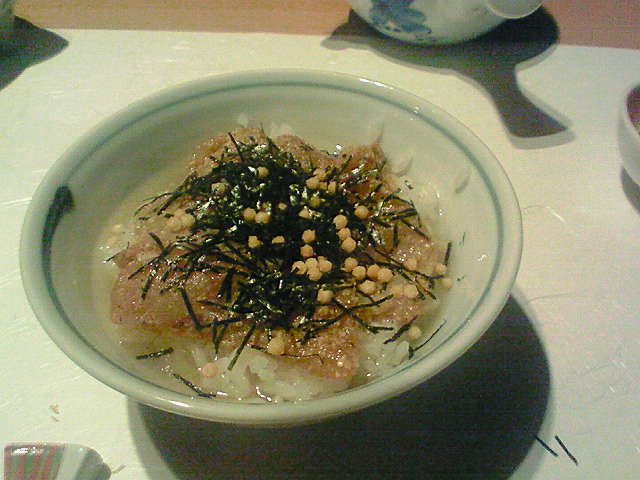In this detailed photograph, a white round bowl with a blue rim sits centrally on a brown table adorned with a white placemat. Inside the bowl, you can see a base layer of white rice topped with pieces of fish and golden corn kernels. The fish appears to be seasoned or sauced, featuring a pinkish-beige hue. A green garnish, perhaps chives, parsley, or rosemary, is artfully sprinkled atop, along with small beige pellets which could be some exotic seasoning or garnish. The bowl is slightly filled with liquid, giving an impression that it might be a soup or a saucy dish.

Surrounding the main dish, various white ceramic items are arranged on the table, including a round white dish to the right of the bowl, and a white ceramic pitcher with a blue design on it positioned behind the bowl. Additional cups, possibly teacups with blue writing, are also visible around the table. Scattered on the table are stringy green leaves, adding a touch of casual detail to the elegant setting, which seems to resemble that of a fancy restaurant.